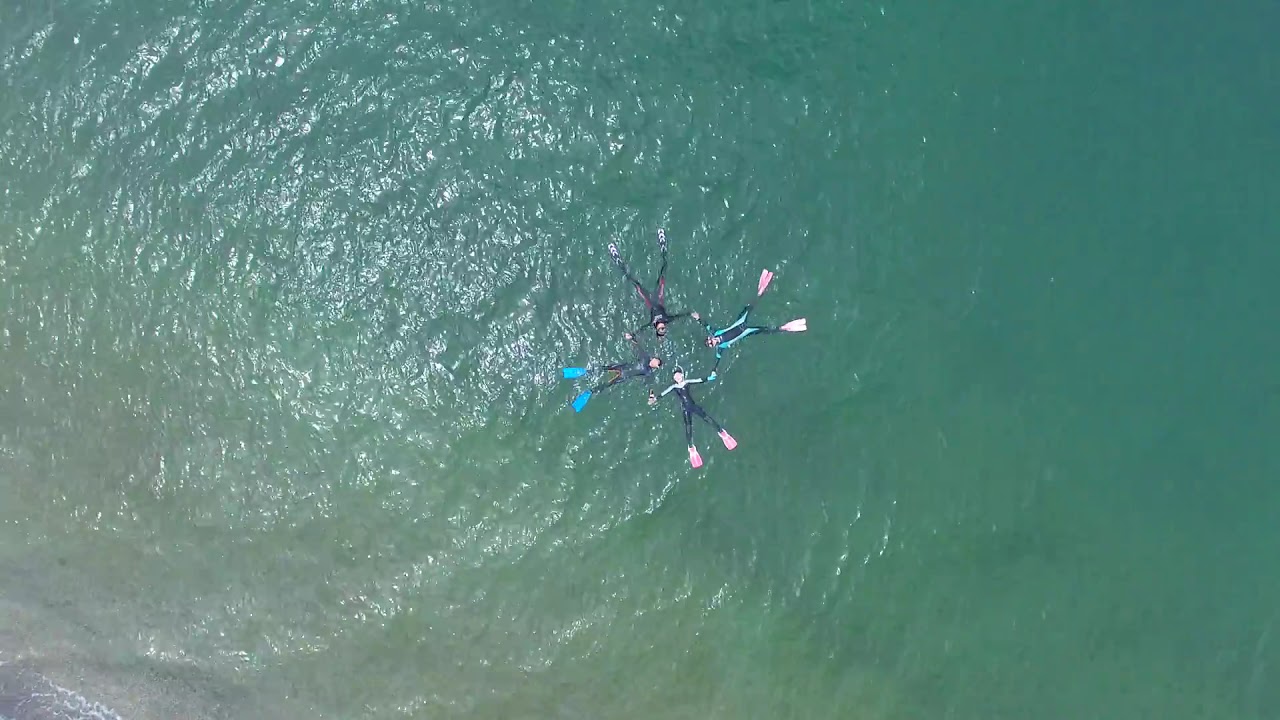This aerial view captures a serene, sunlit scene in a vast body of water, possibly the ocean, with its blue-green hues extending as far as the eye can see. At the center of the image, four individuals dressed in black wetsuits, some accented with green and red, float on their backs in a square formation. Their arms are extended and linked together, creating a cohesive shape amidst the endless expanse of water. Their faces, with pink complexions, are visible as they lie on their backs. The diversity in their flippers adds a splash of color: two wear pink flippers, one has light electric blue flippers, and the fourth has black and white flippers. The overall composition, devoid of any text, is accentuated by the gentle reflections of sunlight on the water, hinting at a clear, sunny day. The aerial perspective, combined with the calm arrangement of the subjects, beautifully encapsulates the tranquility and unity of a shared aquatic experience.